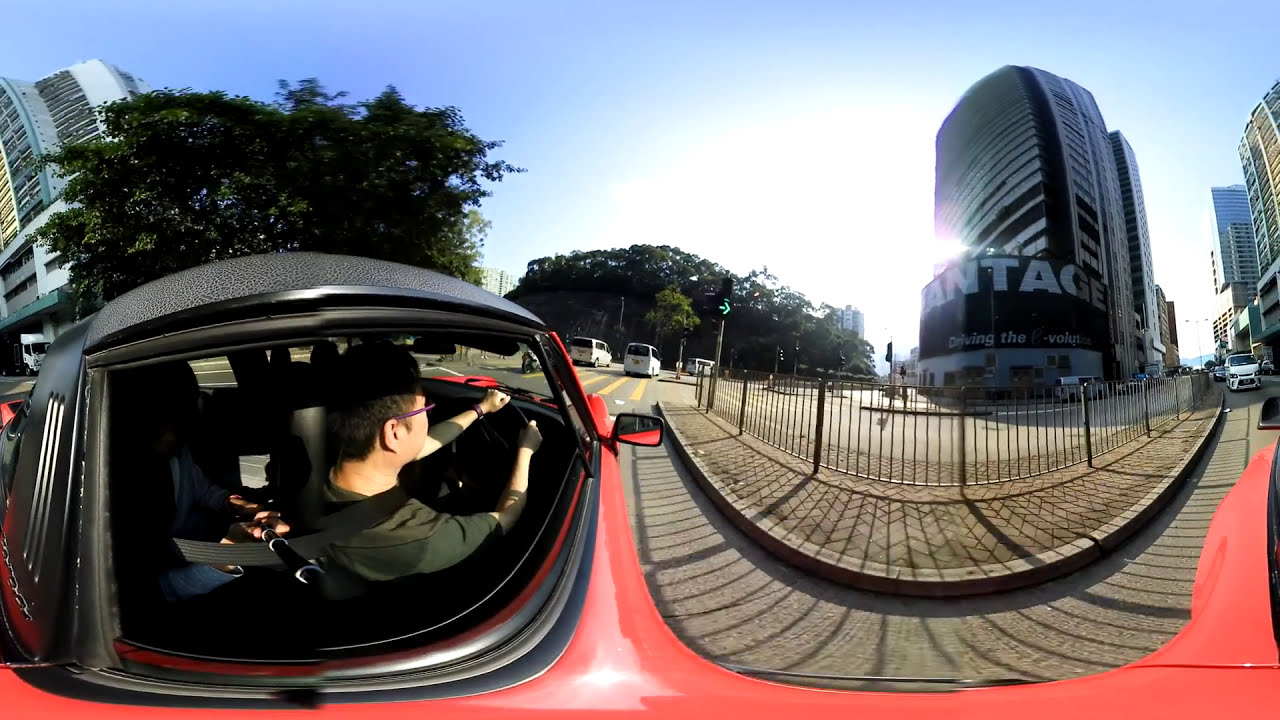A photograph captures a man with short dark hair and glasses, wearing a black t-shirt and a seatbelt, driving a small red car with a black roof. He's steering the vehicle on a curved, U-shaped city street flanked by tall buildings, potentially skyscrapers, that frame the scene on both the left and right sides. The distorted lens creates a double exposure effect, making parts of the image appear warped. To the right of the man, a green arrow on a streetlamp signals go or turn right, and a black metal fence borders the sidewalk. In the background on the left, another person in a blue outfit sits in the back seat. Several white vans are parked in front of a tree-lined area to the left, with a partially obscured building sign visible, displaying the letters "A-N-T-A-G-E." The scene is bathed in soft sunlight under a light blue sky.